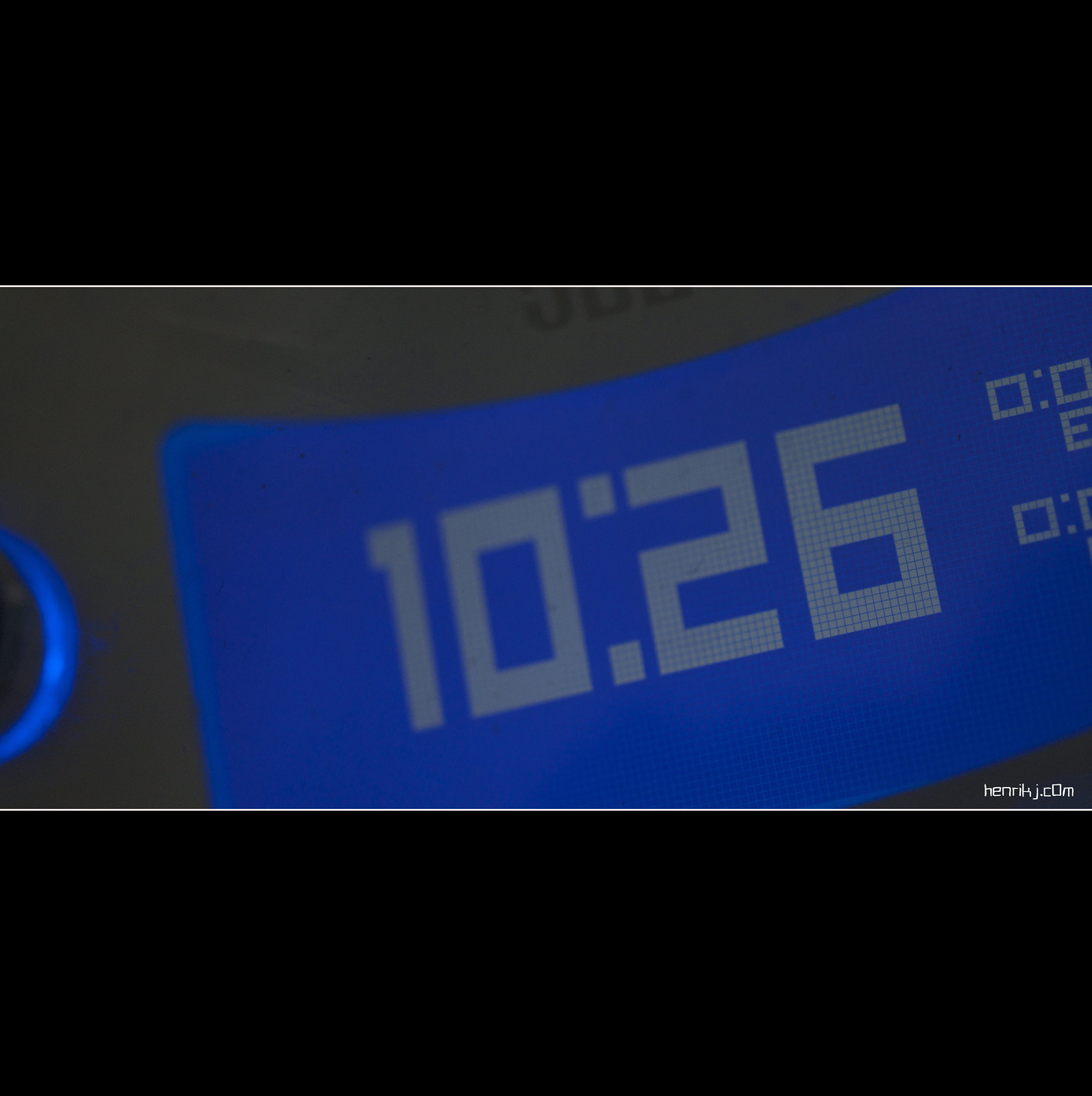The image displays a horizontally-oriented alarm clock LCD screen set against a black background, framed by black bars on both the top and bottom. In the center of the image, the LCD screen is divided from the black borders by thin white lines. The LCD screen itself has a gray background and shows the time "10:26" prominently in a gray tone on a blue surface. Toward the right side of the bottom portion of the screen, the text "h-e-n-r-i-k dot j dot c-o-m" is visible, suggesting a website or signature. The clock screen slightly curves from the edges to the center. To the left of the screen, there appears to be a partially visible twistable knob or joystick with a blue LED forming a ring underneath it. This additional element hints at the device's adjustability or additional functionalities.